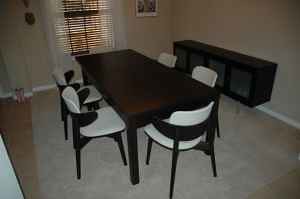This color photograph depicts a small dining room with tan walls and a floor that is a light brown, possibly linoleum or hardwood. Centrally featured is an oblong, dark wood dining table, surrounded by five chairs. The chairs are distinctive with their white seats and backs, framed in black with black legs. The table is arranged longitudinally from near a window on the left wall towards the lower right corner of the image. The window has white trim with blinds that are nearly closed, allowing just a sliver of sunlight to seep through. On one of the walls, a dark brown sideboard adds an elegant touch to the room. Additionally, there is a door in the background with a small window dressed with narrow Venetian blinds. Further back on the walls, a couple of pictures add to the decor, though their details are indistinct from this angle. The entire area is draped in subtle shadows, contributing to its cozy and intimate atmosphere.